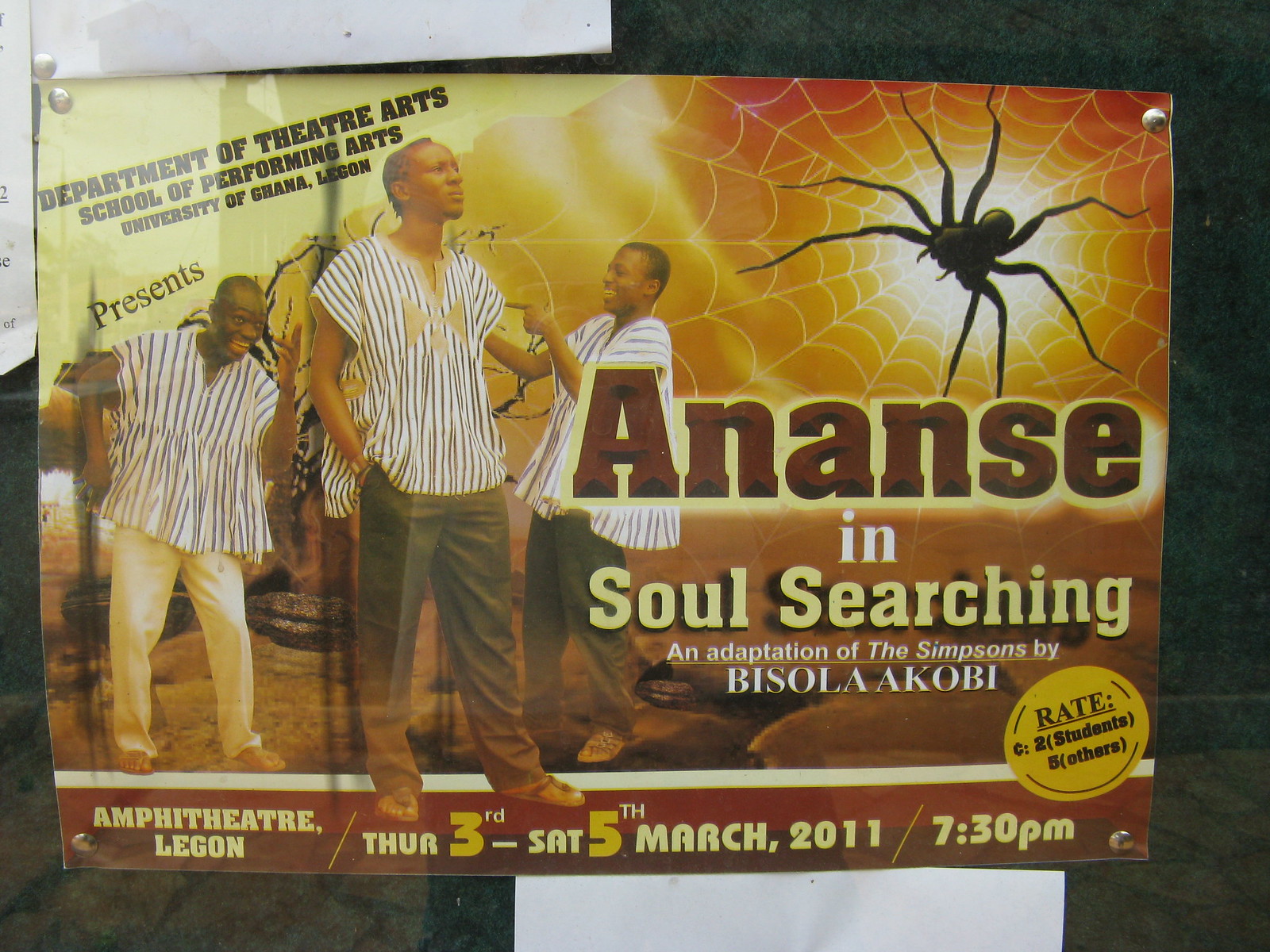This detailed photograph captures an advertisement pinned up against a reflective dark green or black board with patches of white. The advertisement itself features a prominent orange background with a striking black spider situated in a web in the top right corner. Above the spider, the sign reads, "Department of Theatre Arts, School of Performing Arts, University of Ghana, Legon." Below this heading and to the left of the spider, three men dressed in black and white dashikis are depicted. The man in the middle, the tallest, gazes upward while flanked by two dancers, one to his left looking downward, and another to his right pointing towards him. Two of the men wear dark brown pants while the third is in light brown pants.

The text on the right side of the advertisement presents "ANANSE," in bold letters, followed by "Soul Searching, an adaptation of The Simpsons by Bisola Akabi." The bottom section of the advertisement, covered by a red banner, details the event's specifics: "Amphitheatre Legon, Thursday 3rd to Saturday 5th March 2011, 7:30 PM." A yellow circle indicating the admission rates, reading "Rate C, two students, five others," is also visible on the bottom right. The scene appears to be captured outdoors, hinting at an early evening setting based on the reflective surface and subtle lighting. The colors in the advertisement range from white, black, and grey, to shades of yellow, orange, red, and tan, adding to the visual appeal of the image.